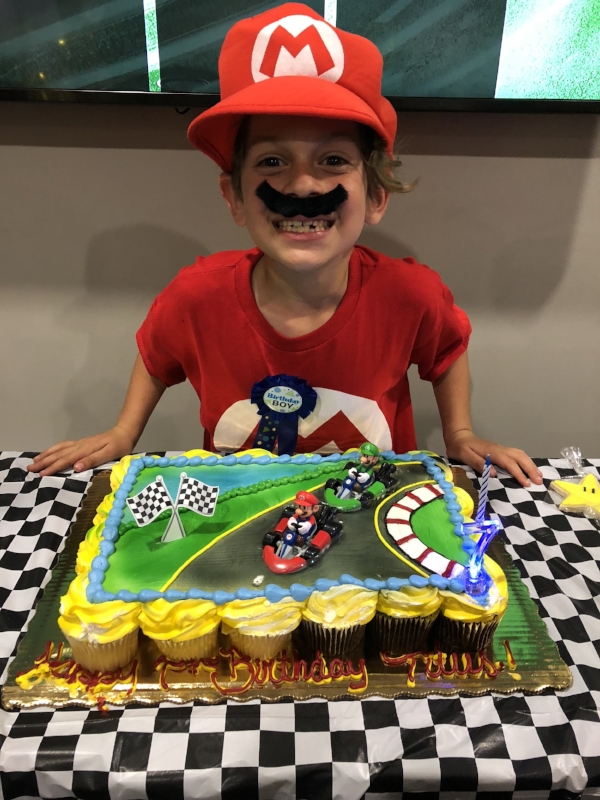This photograph captures a joyful boy at his Mario-themed birthday party. He is wearing an oversized foam Mario cap with the iconic red "M" emblem, a red Mario t-shirt featuring the same symbol, and a fake black mustache. His dark brown hair peeks through the cap, and a blue ribbon, declaring "Birthday Boy," is pinned to his shirt. The boy, named Titus, is standing in front of a Mario Kart-themed cupcake cake, topped with race cars of Mario in the lead and Luigi following on a vibrant racetrack design. The text on the cake reads "Happy 7th Birthday Titus!" with an exclamation point. The festive black and white checkered tablecloth mirrors a racing flag, and a star-shaped cookie wrapped in cellophane is visible to the side, enhancing the Mario theme. Titus looks thrilled, embodying the excitement of his special day.